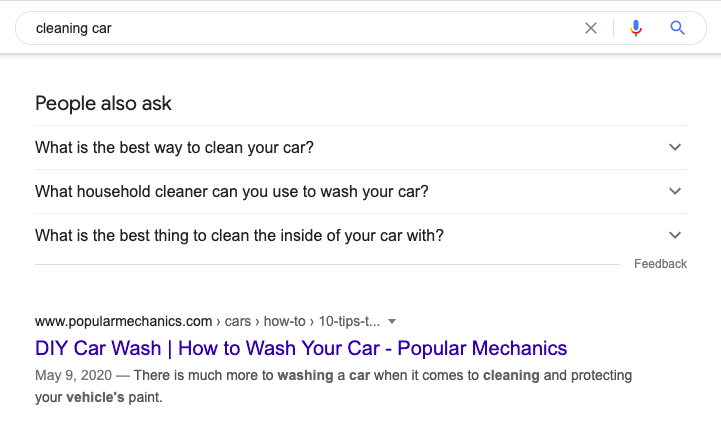This image displays a search results page centered around the query "cleaning car." In the search input field, the phrase "cleaning car" is clearly visible. To the right of the input field are three buttons: the "clear" or "delete" button, the "voice input" button, and the "search" button.

Below the search bar, the "People also ask" section is prominently featured, showcasing related questions such as "What is the best way to clean your car?", "What household cleaner can you use to wash your car?", and "What is the best thing to clean the inside of your car with?".

Further down, a highlighted search result from www.popularmechanics.com appears. The result includes a link to an article titled "DIY Car Wash: How to Wash Your Car," published on May 9, 2020. The snippet of the article emphasizes the importance of comprehensive car washing, noting that there is much more to it when it comes to cleaning and protecting your vehicle's paint.